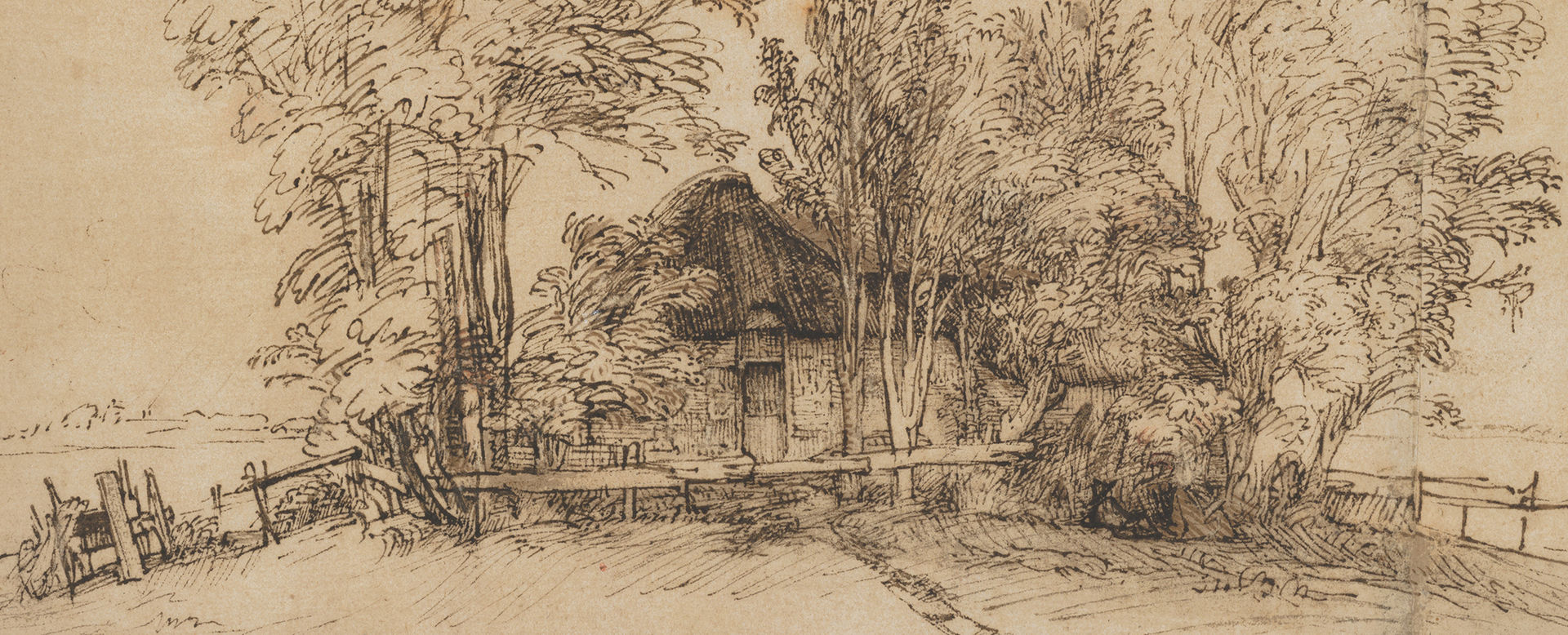This sepia-toned drawing depicts a rustic cabin with a thatched straw roof prominently placed at the center. The cabin is surrounded by an array of large, leafy trees, providing ample shade and creating a serene backdrop. A well-defined pathway leads from the front door of the cabin to the bottom edge of the image, suggesting an inviting route towards the abode. On the right side of the house, a small wooden fence is seen, potentially serving as a boundary or decorative element. Adjacent to the left of the cabin, there appears to be a carriage-like object, adding to the rustic ambiance. The ground in front of the house is cleared and flat, contributing to the orderly arrangement of the scene. Overall, the drawing exudes an earthy, nostalgic charm with its predominant shades of brown, capturing the essence of a peaceful, secluded woodland retreat.